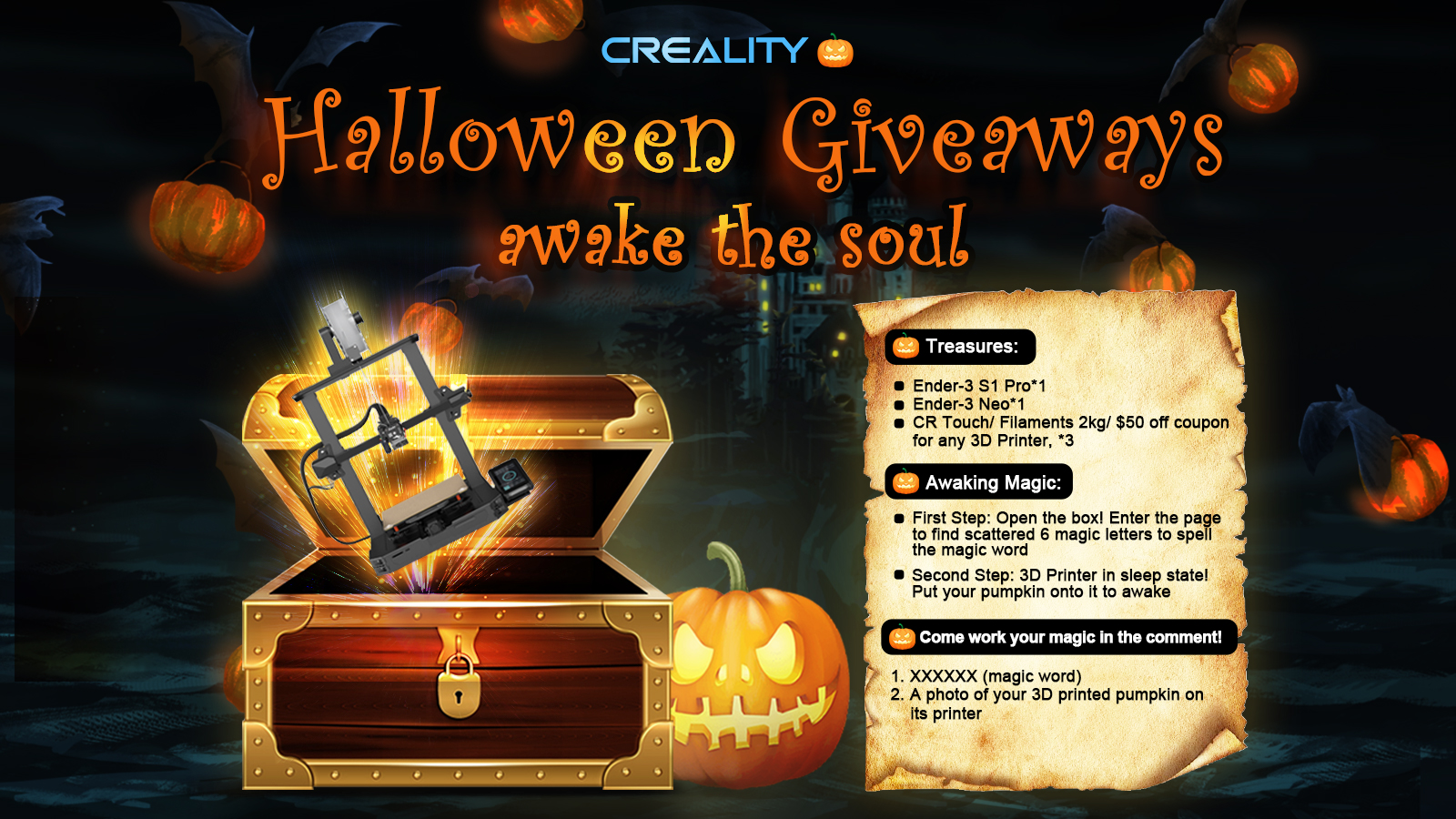The image is a vibrant Halloween-themed promotional banner from Creality, featuring an array of festive elements. Dominating the top portion is the text "Creality" in bold blue letters, with "Halloween Giveaways Awake the Soul" written below in bright orange. The central area showcases six floating orange pumpkins, adding a playful touch to the dark, eerie ambiance.

At the bottom left of the screen, an open treasure chest, adorned with gold framing, spills out a curious gray object. Next to it, a carved pumpkin emits a warm yellow glow, casting an inviting light and adding to the Halloween spirit. To the right, a piece of parchment lists three intrigue-filled categories: "Treasures Awake," "Magic," and "Come Work Your Magic in the Comments." Each section contains various notes, enticing viewers to participate.

The background is a haunting mix of dark gray and black hues, enhancing the spooky atmosphere. In the distance, a shadowy house with flickering yellow lights peeks through the darkness, adding a mysterious element. Finally, the top left corner is adorned with bat designs, completing the quintessential Halloween scene.